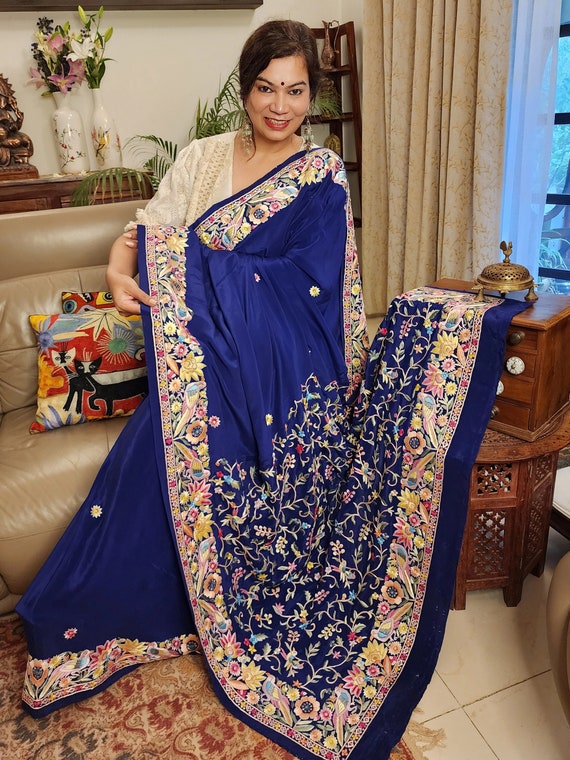The photograph depicts a woman standing in a living room adorned with off-white and beige decor. She has dark, short hair styled into a bun pulled to the side, and she wears long, ornate earrings. A distinctive dot graces her forehead between her eyes, hinting at cultural or religious significance. Her attire is a striking royal blue sari with a heavily embroidered floral border that features intricate flower petals connected by ivy. The sari drapes elegantly, revealing a light, likely ivory-colored blouse underneath. The room itself is decorated with ivory-colored draperies, an ivory leather couch, and an ivory tiles floor. The walls are a soft off-white, with a window on the right featuring tan curtains. A rug lies on the floor, and decorative pillows adorn the couch. There are also flowers in vases on a side table, adding to the serene ambiance of the space.